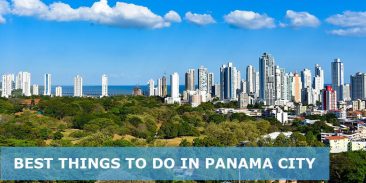A stunning photograph captures the scenic beauty of Panama City, set against a brilliant blue sky adorned with white clouds. The cityscape features a multitude of tall buildings, indicative of a bustling downtown area filled with office structures and hotels. In the foreground, there's an open space characterized by rolling hills and lush greenery, which suggests a park-like setting. The azure sea forms the backdrop, enhancing the visual appeal of the image. A prominent blue banner with white lettering at the top reads, "Best Things to Do in Panama City," hinting that the photo might be sourced from a website or travel guide. The image beautifully showcases the juxtaposition of urban and natural landscapes, highlighting Panama City's allure.